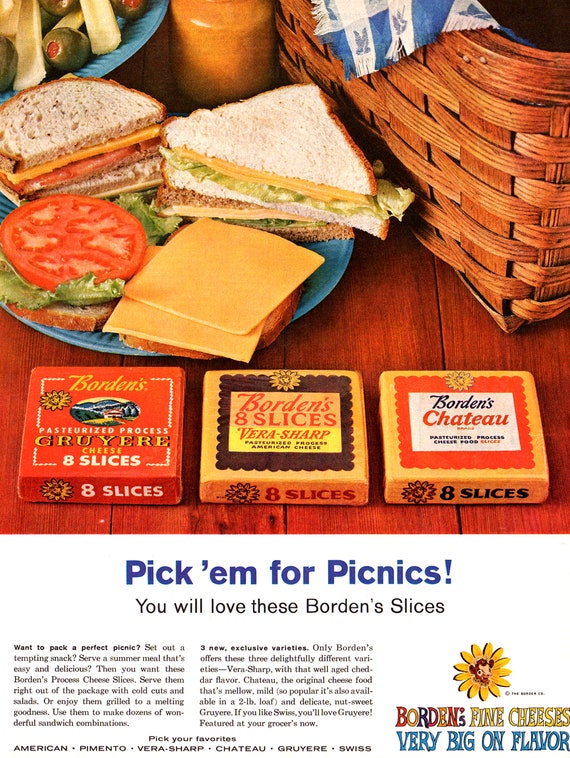This old-fashioned advertisement for Borden's cheese, seemingly from the 1960s or 1970s, captures a nostalgic picnic scene. At the top of the image, a blue and white checkered cloth spills from a brown wicker picnic basket. To the left, a blue plate displays a sandwich cut in half, showcasing layers of cheese, tomatoes, and lettuce. An open-faced sandwich sits nearby, revealing slices of cheese and lettuce. In the top left corner, a bowl filled with olives and celery adds a touch of variety.

Dominating the lower portion of the advertisement, three different types of Borden's cheese are prominently featured. Each package contains eight slices and boasts unique packaging. The leftmost variety is encased in a red wrapper, while the middle cheese has a black center label surrounded by an orange exterior. The rightmost cheese is presented in clear packaging with a red label.

Text at the bottom encourages viewers to "Pick'em for Picnics," highlighting the appeal of Borden’s slices for outdoor gatherings. Additional text in the bottom right corner emphasizes the product's quality with the slogan, "Borden's fine cheese is very big on flavor," accompanied by a whimsical symbol of a cow centered in a sunflower. Each paragraph further describes the attributes and flavors of the cheeses, reinforcing the brand’s promise of delightful picnic fare.